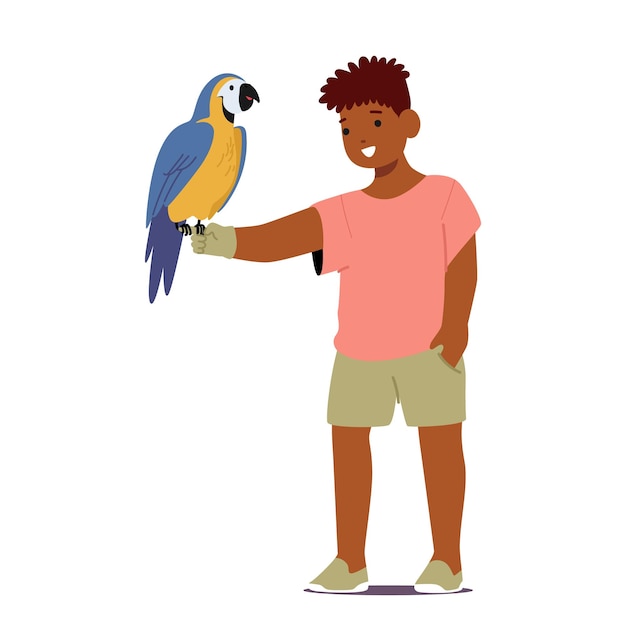The illustration depicts a young boy with a medium-dark skin tone, brown poofy hair, and simple facial features that include brown eyebrows, two small black dots for eyes, a tiny line for a nose, and an open mouth shaped like a white half-circle. He is dressed in a pink crew neck t-shirt paired with beige pants and beige shoes that have white soles. The boy stands on a surface casting a shadow in the form of a purple circle. His left hand rests in his pocket while his right arm extends to the left, adorned with a glove holding a vibrant blue and yellow Macaw. The bird features a white face and a black beak, with a bright yellow belly and blue feathers extending from the top of its head down through its wings and tail. The background of the image is stark white, enhancing the vivid colors of the characters. This scene resembles a piece of clip art or digital illustration characterized by its simple, bold graphics.